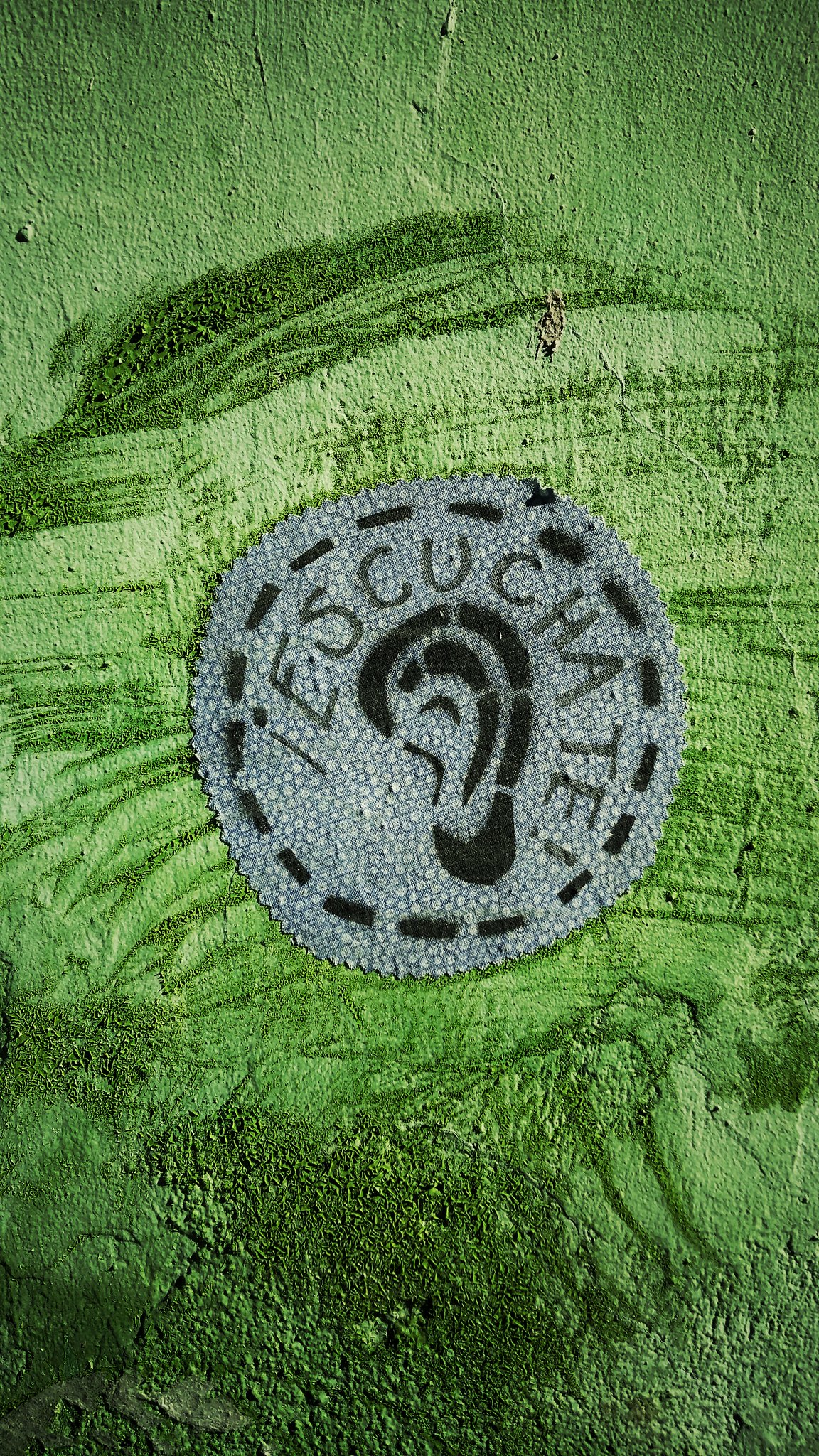The image is a detailed, portrait-oriented color photograph, enhanced through illustrative and filter techniques. The backdrop is a wall painted in various shades of green, characterized by a rough, cracked texture with visible horizontal brushstrokes and vertical patches near the bottom. Central to the image is a circular, gray object with the surface resembling a pebble. This gray circle features a black, spray-painted stencil image with a dotted broken line around its outer edge. At the center of the gray object, an ear outline is drawn, also spray-painted. Surrounding the ear, the phrase "escúchate!" is inscribed in a circular formation, written in black marker. The overall style of the artwork combines elements of color photography, illustration, and specialized filters.